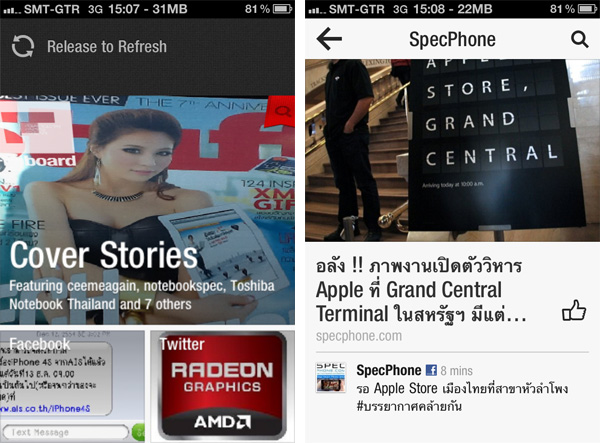**Detailed Descriptive Caption:**

The image showcases two juxtaposed screenshots, each seemingly representing a smartphone interface with varied content.

**Left Screenshot:**
- **Signal/Battery:** The top bar indicates a signal strength of three out of five bars, labeled as "SMT GTR 3G 1507." The numeric value "-31 MB" is displayed alongside an 81% battery indicator. A refresh icon appears with the message "Release to refresh."
- **Content Overview:** 
  - **Magazine Cover:** Prominently features a woman on a magazine cover, the headline proclaiming "Cover Story featuring Key Megan." Additional titles include "Those Notebooks Back, Time to Shiva Notebook," and references to "seven others."
  - **Social Media:** 
    - **Facebook:** Toward the bottom section, there are Facebook-related elements, including a section that appears to contain a tirading text message and an old-style iPhone graphic.
    - **Twitter:** Another box situated at the bottom right contains Twitter-related content, with a mention of "Twitter rating and graphics." The text "D and I" and "graphics card" appears within this section.

**Right Screenshot:**
- **Signal/Battery:** Similarly, the top bar shows a signal strength of three out of five bars, labeled "SMT GTR 3G 1508," with "-22 MB" and an 81% battery indicator.
- **Content Overview:** 
  - **Image:** Features a person on a staircase next to a signboard labeled "Grand Central."
  - **Text and Icons:** 
    - **Apple Branding:** The text "Apple" is interspersed with Thai writing, repetitive mentions of "Grand Central terminal," and a thumbs-up symbol.
    - **Web Reference:** Labelled "specphone.com."
    - **Navigation Bar:** Displays a gray bar running horizontally.
    - **Social Media:** 
      - **Facebook:** There is a blue box with a picture, possibly linking to "specphone" and the Facebook symbol. There is a mention of "eight minutes" in context with Thai writing. The rest of the screen contains similar Thai script against a gray background.